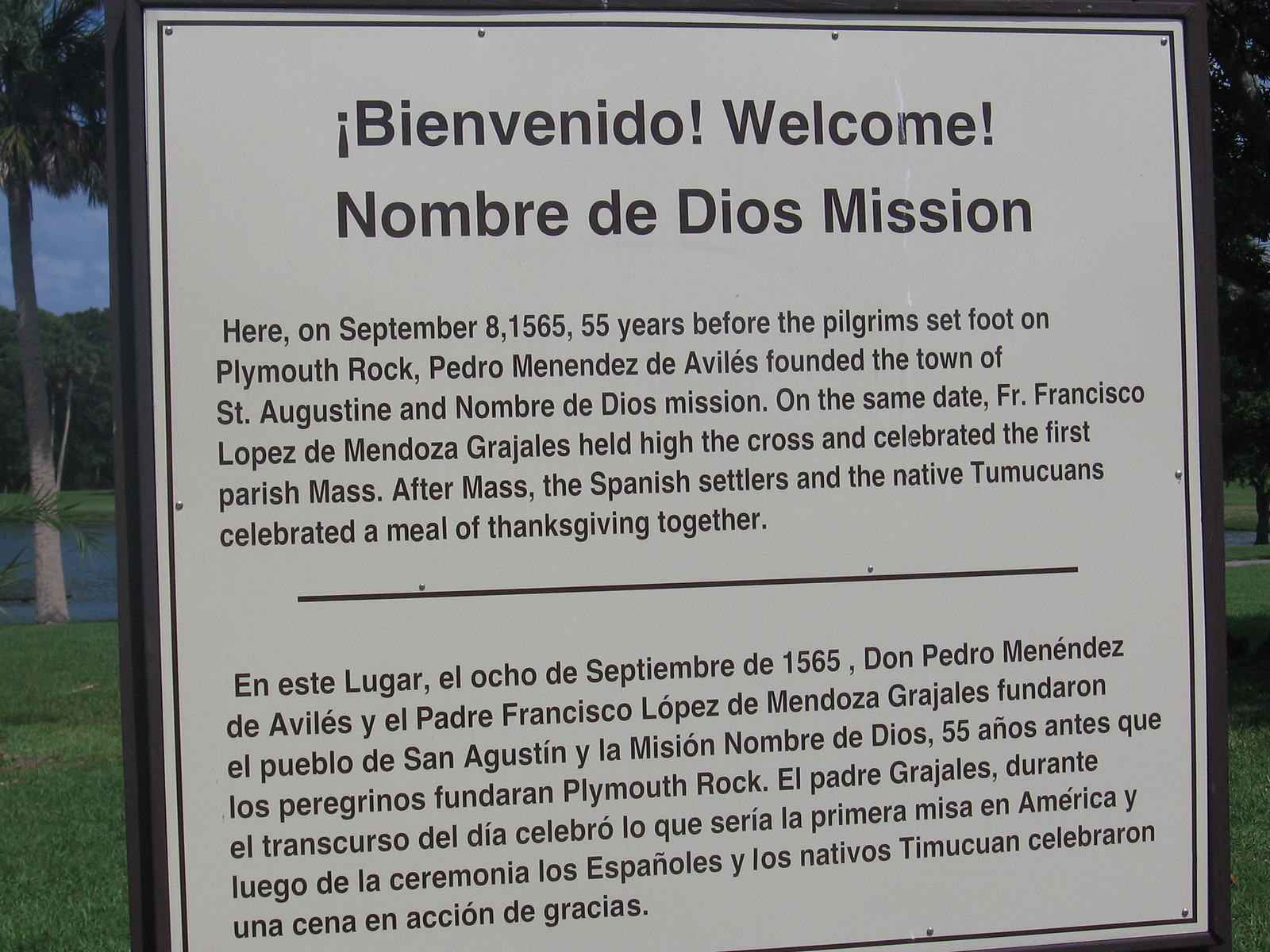A photograph depicts a historical marker inside a building, viewed through what appears to be a glass window. The sign welcomes visitors in both English and Spanish. Based on the sign, the location is identified as St. Augustine, Florida. The sign design does not appear professionally done and looks somewhat like it could be Photoshopped onto the image. It lacks the polished appearance typical of official historical markers, suggesting it might have been created by a private property owner rather than an authoritative historical organization.